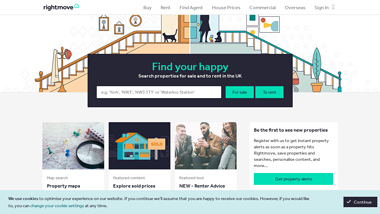**Website Screenshot Description: Rightmove Real Estate Platform**

This is a screenshot of a webpage, which appears to be a real estate website, likely Rightmove based on the context. However, the exact URL is not displayed. The top navigation bar contains the following links: Buy, Rent, Find Agent, House Prices, Commercial, Overseas, and Sign In.

Below the navigation bar, two side-by-side images create a split view of an indoor and outdoor setting. The left image showcases the inside of a home with a staircase. At the top of the stairs is a platform, and visible on the left side are a cat, some pictures hanging on the wall, and a banister leading down to the left. At the bottom of these steps is a coat rack with a hat and a jacket.

The right image portrays an outdoor scene featuring silhouettes of an adult and a child. The child appears to be playing with stacking blocks. The banister this time leads the stairs down to the right, ending near a potted plant with a single leaf. There's an obscured object that is partially visible in front.

Centrally located on the page is a black search box which prompts users to "Search properties for sale and to rent in the UK" followed by the tagline "Find your happy." The search box includes alphanumeric examples likely representing location or postcode searches, with options for "For Sale" and "To Rent."

Below this, there is a block of three images:

1. **First Image**: Features a map with pushpins, a magnifying glass, and a partially visible spiral-bound notebook. Text is present but not legible, with a caption reading "Property Maps."

2. **Second Image**: Depicts a simple illustration of a two-story house with a green exterior and orange roof. A "Sold" sign is posted out front. The caption underneath reads "Explore Sold Prices."

3. **Third Image**: Shows three individuals, including two male-presenting figures and one female-presenting figure. The central figure appears to be on their phone. The accompanying text mentions the words "New" and possibly "Renter" and "Advice."

Adjacent to these images, on the right side, there is a white box with a header that seems to say "Be the first to see new properties." This box contains a green link prompting users to "Get property details or alerts," though the exact wording is not entirely clear.

Finally, at the bottom of the page is a footer box related to cookie consent. The text in this footer is not legible, but it includes a link that turns green against black text. There are checkboxes and a "Continue" button towards the far right. The footer is designed within a black box on a light green banner.

This detailed description captures the essence and layout of the website as presented in the screenshot.